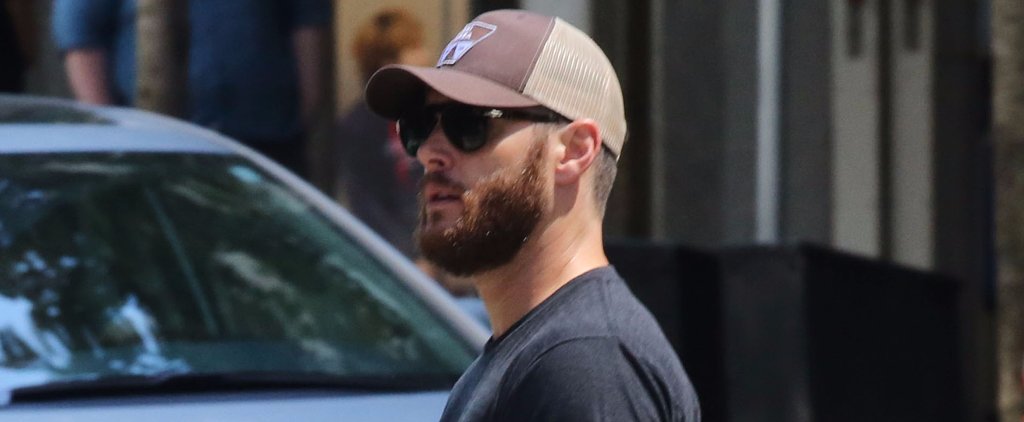The photo captures a side view of a man in his 30s with a short brown beard and black sunglasses, facing the left. He is wearing a brown cap with a white plastic backing that has small holes, and a black shirt visible up to just below his shoulders. His ears are slightly red, and he has short hair visible below the cap. The lighting comes from the upper right, casting shadows on his left side.

In the background, on the left side, there is a slightly out-of-focus white or silver car with a dark sunroof, showing its windshield and part of the hood. You can see the edges of a gray building on the right. Behind the man, off in the distance, there is a person with light brown hair facing a store door or wall. This person is accompanied by a child with medium-length brown hair, wearing a long-sleeved black shirt with a red logo. Both stand close to a skinny tree trunk. The multiple buildings in the background are blurred out.